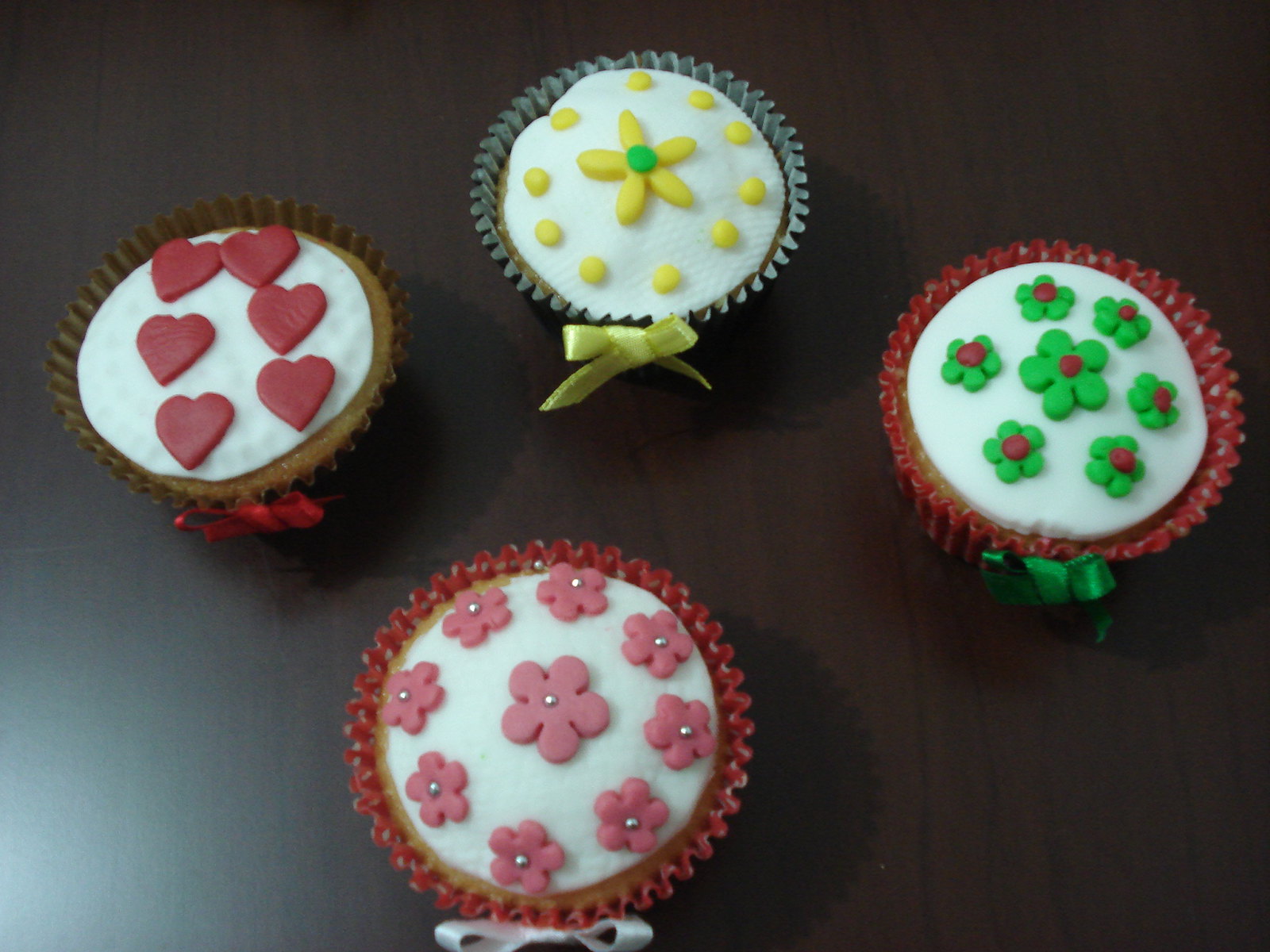This top-down photograph captures four meticulously decorated cupcakes, arranged in a diamond pattern on a mahogany brown tabletop. Each cupcake features intricate designs that go beyond typical frosting, embodying the artfulness found in high-end cakes.

- On the left, a cupcake sits in a brown wrapper with a red ribbon. It has white frosting adorned with six red fondant hearts arranged vertically.
- At the top, a cupcake in a green wrapper with a yellow ribbon showcases white frosting with yellow polka dots arranged in a circle, centered by a yellow flower with a green middle.
- To the right, another cupcake in a red wrapper with a green ribbon is decorated with green floral designs on white frosting, each flower featuring a red center.
- At the bottom, a cupcake in a red wrapper with a white ribbon displays white frosting topped with pink flowers, each flower highlighted by a silver dot in the middle.

The attention to detail in the decorations, from the colorful designs to the carefully chosen ribbons, elevates these cupcakes into miniature works of art.